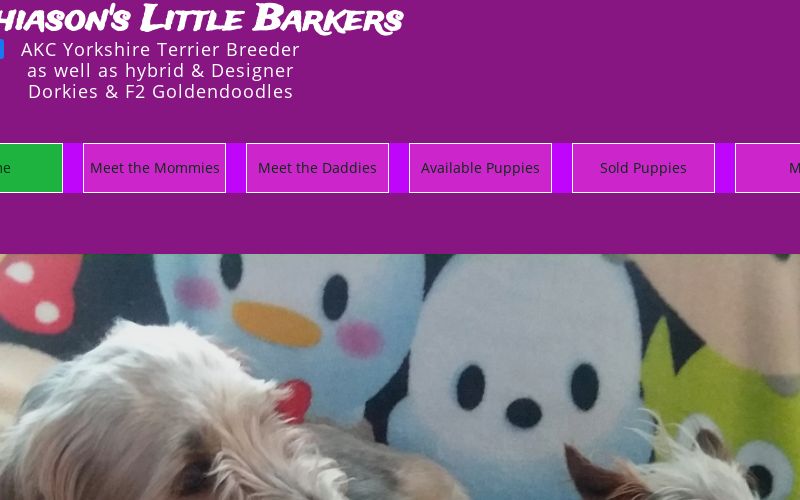The advertisement page features a prominent purple heading with "HIASON'S Little Barkers" written in bold white capital letters. Below this heading, it reads "AKC Yorkshire Terrier Breeder" followed by "Hybrid and Designer Breeds: Dorkies and F2 Golden Doodles." This text is placed above a green box, partially visible, showing the letter 'E' in black.

Adjacent to this green box, the page has a section with light purple backgrounds containing black-lettered titles: "Meet the Mommies," "Meet the Daddies," "Available Puppies," and "Sold Puppies." Another purple box appears alongside these titles, but only the letter 'M' is visible due to cropping.

The lower section of the page features a purple border and a partially visible image of two puppies. The one on the right shows only its ears and the top furry part of its head, while the puppy on the left reveals its right eye surrounded by long, white fur. The background includes whimsical elements such as a face with black eyes and a black nose, another face with two black eyes, two pink cheeks, and an orange nose, and an image resembling Minnie Mouse adorned with a red bow and white polka dots.